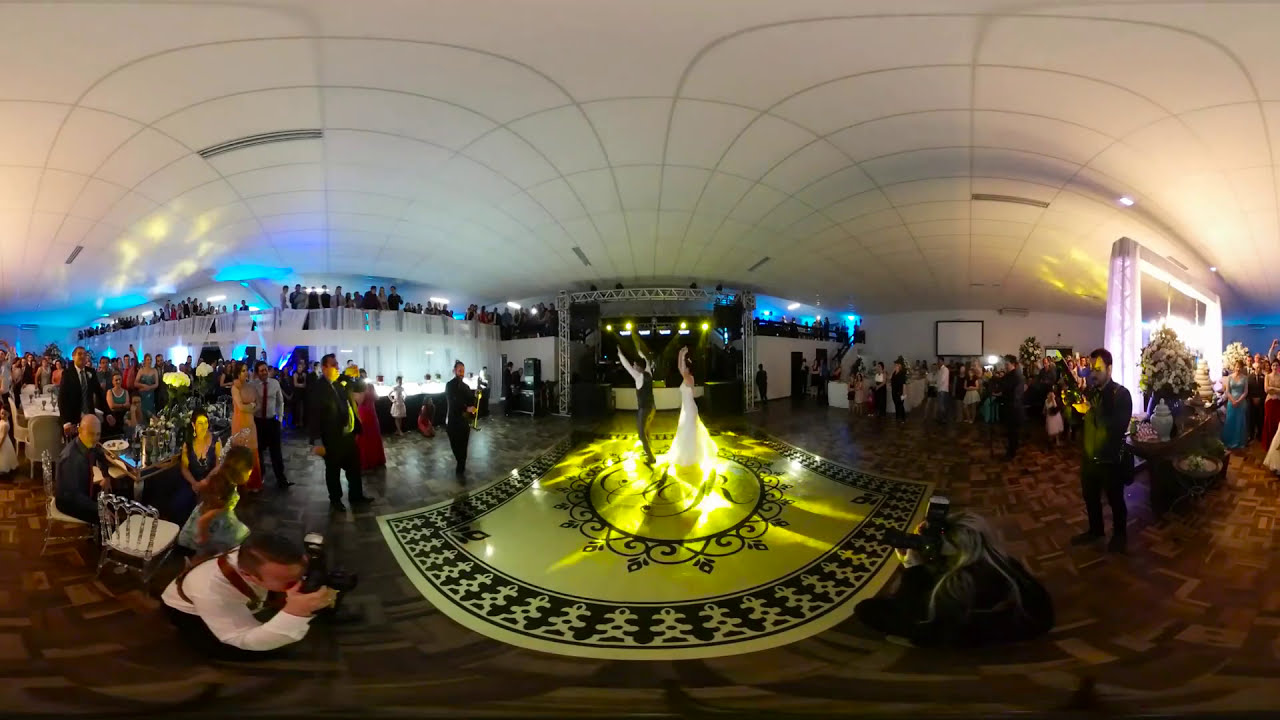This panoramic image captures the vibrant scene of a wedding reception held in a spacious ballroom. The room features a white ceiling and dark brown parquet flooring. In the center, the bride and groom are the focal point, dancing joyfully on a distinctive, ornate black-and-white scroll-patterned rug. The groom is dressed in a black vest over a long-sleeved white shirt, while the bride wears a long, white gown with an accessory in her black hair. Both have their arms raised in the air, a gesture echoed by the festive mood of the occasion.

Bright yellow lights illuminate their feet, adding a warm glow to their dance floor. Surrounding this central area, guests in dresses and suits are either seated at tables or milling about, many capturing the moment with their cameras. Some photographers are even seated on the ground to get the perfect shot. The image also reveals a balcony in the background, filled with more guests, illuminated by subtle blue lights. On the right side of the image, a large bouquet of flowers adds to the décor, and a stage is visible in the distance, though it appears unused at this moment. The overall atmosphere is one of celebration and elegance, beautifully framed by the grandeur of the ballroom.